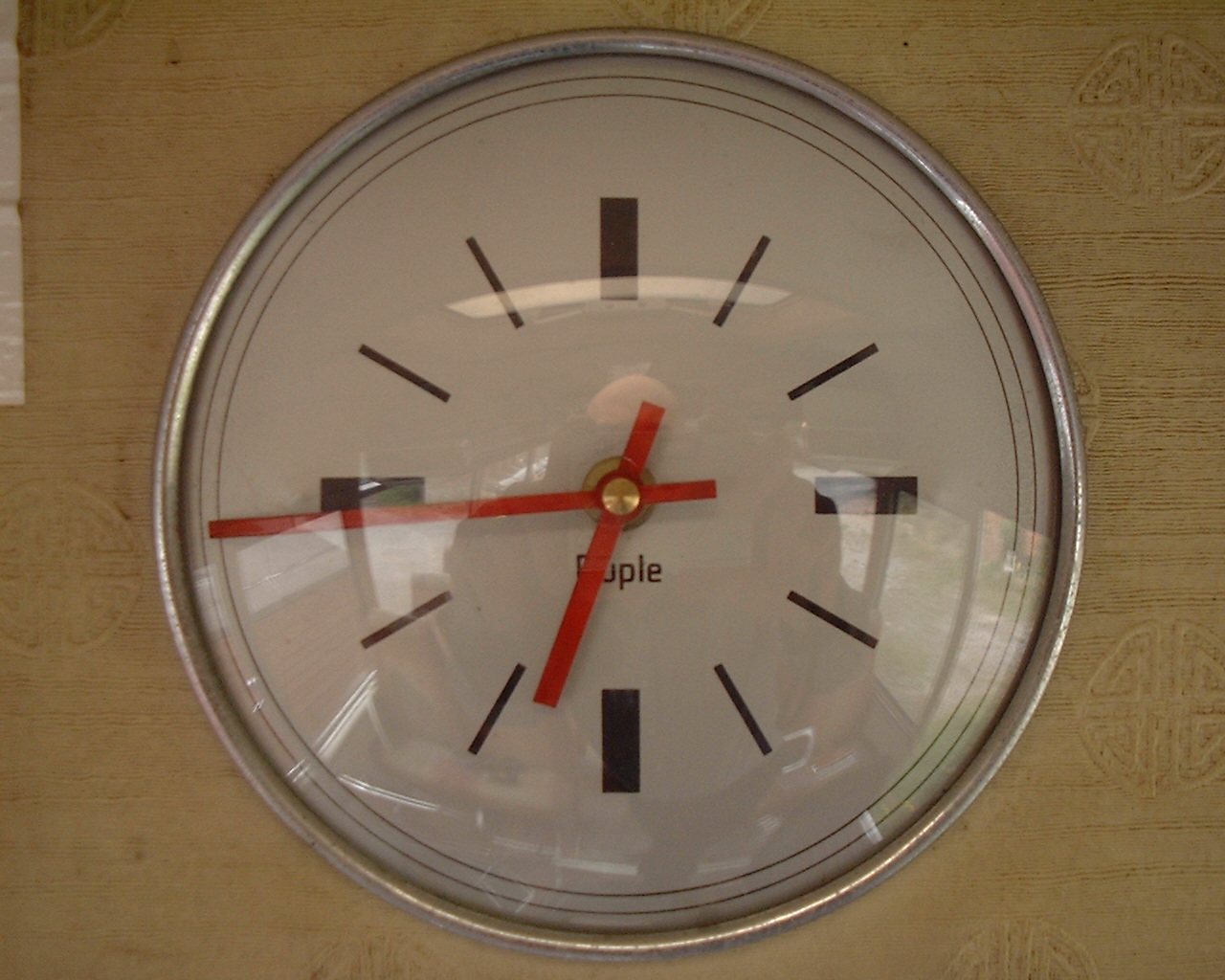A round wall clock with a sleek, shiny silver frame is displayed against a textured beige wall. The wall is adorned with subtle, raised insignias showcasing circular patterns with crosses at their centers. The minimalist clock face is devoid of numbers, featuring only sleek hour markers. Thick lines mark the 12, 3, 6, and 9 o’clock positions, while thinner lines denote the remaining hours. Two striking red hands indicate the time, which is approximately 6:45.